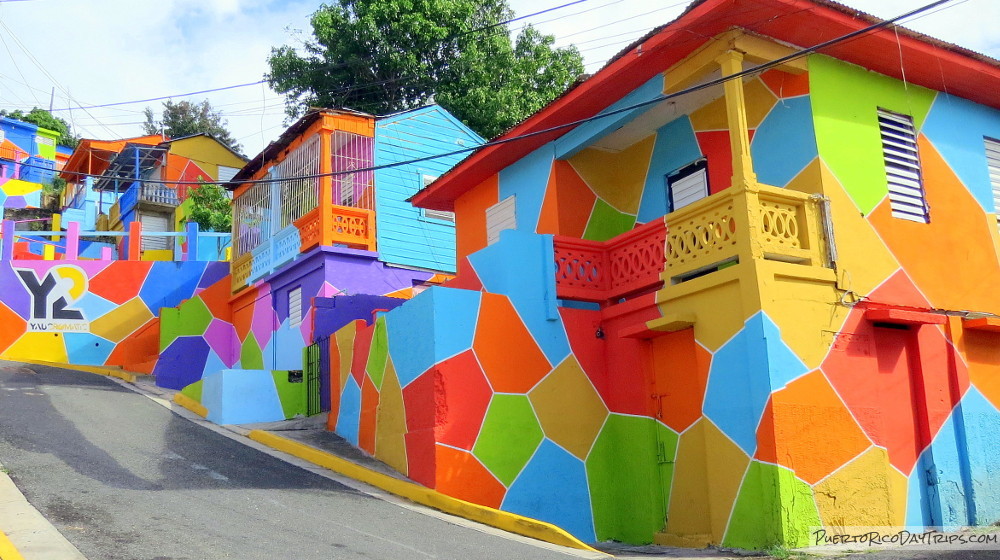This photograph captures a vibrant and colorful hillside street scene, likely in Puerto Rico, characterized by an array of vividly painted houses. The narrow, horizontal image showcases a steep, winding street lined with a yellow concrete barrier on the left. To the right, facing the street, stand approximately six two-story homes adorned with bright, mosaic-like splotches in a palette of orange, yellow, light blue, green, pink, and gold, all outlined in white. The roofs, porches, and even the undercarriages of the roofs are similarly painted, creating a cohesive, multicolored spectacle. The homes feature small patios and balconies, contributing to the tropical ambiance, enhanced further by lush green trees visible behind and above the houses against a backdrop of blue sky and clouds. Power lines stretch across the photograph from the upper right to the upper left, intersecting with the vibrant scene below. On a wall near the top of the street, the label "Y2" is prominently displayed, with additional words beneath it. The photo also prominently displays the URL "PuertoRicoDayTrips.com" in the bottom right-hand corner, suggesting the image is part of a travel promotion.